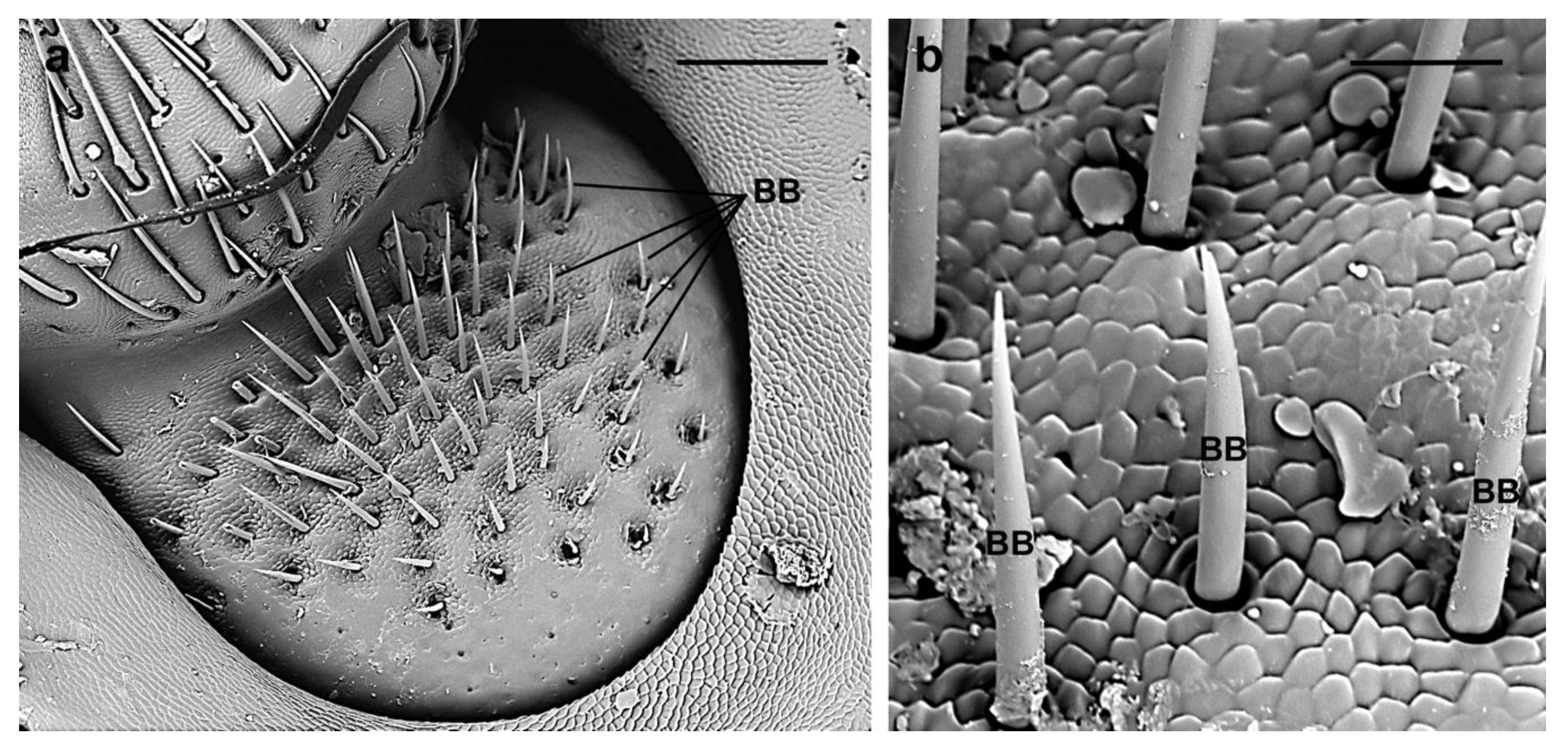These two black-and-white photographs display surfaces with spikes or needle-like structures, seemingly taken under a microscope or extreme magnification. The image on the left, labeled with a lowercase 'a' in the top-left corner, shows a broader view of a textured surface from which these sharp, fang-like protrusions emerge. This surface could belong to a biological or synthetic entity, though it's unclear whether it represents animal cells, plant structures, or something entirely different. The image on the right, marked with a lowercase 'b' in the top-left corner and further labels 'BB' pointing to the spikes, offers an even more magnified view of the same scene, emphasizing the intricate details of these white spikes. The overall layout and labeling suggest a scientific context, potentially a study of hair follicle regrowth or microscopic examination of spiky surfaces.